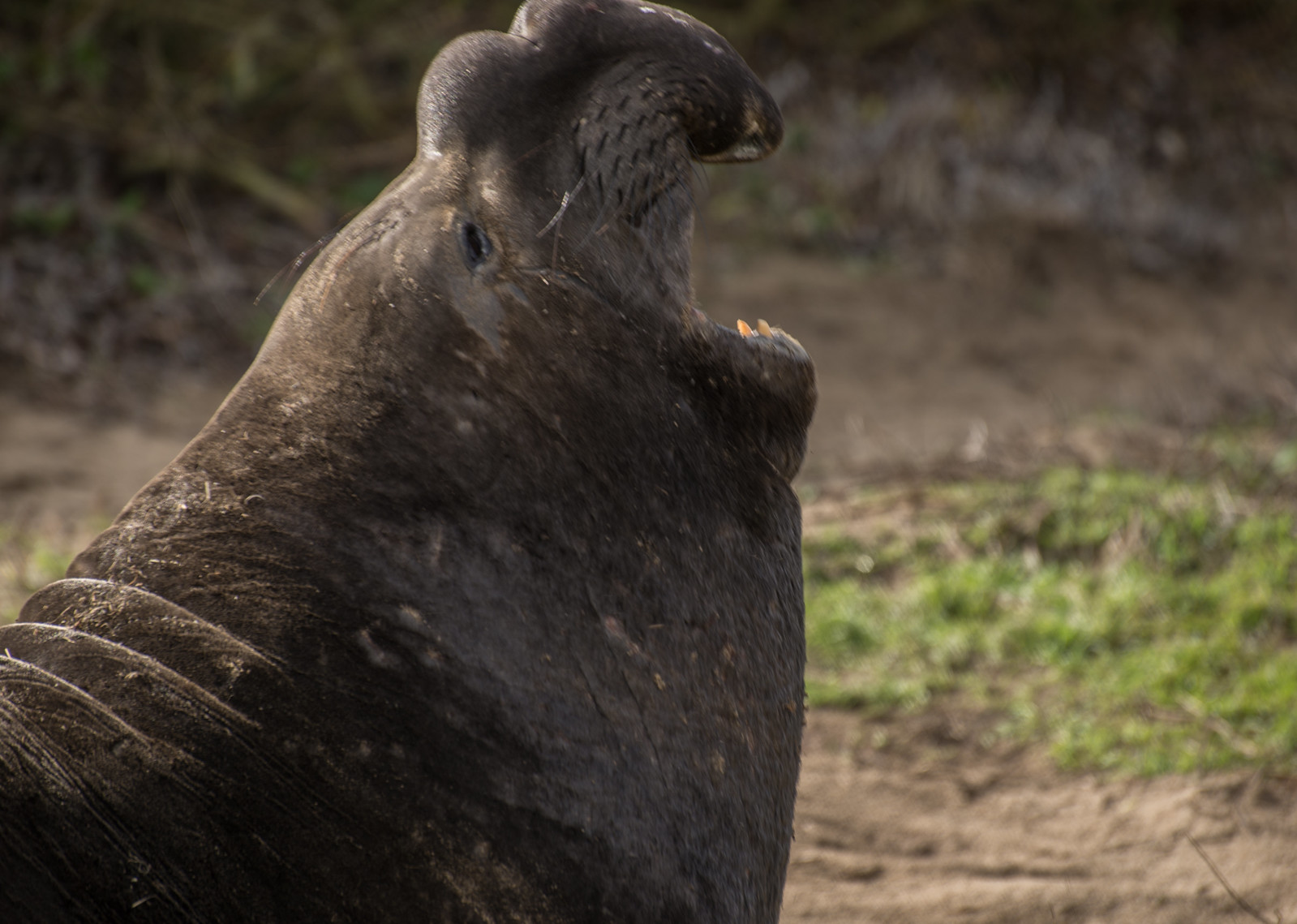This image captures a large seal, potentially an elephant seal, either in its natural habitat or a zoo setting. The seal, featuring a distinctive brown fur adorned with natural lines, dominates the lower left portion of the frame, stretching towards the center. Its characteristic elongated trunk-like nose, curving downward like the shape of the number three, is a prominent feature. With its mouth wide open, the seal appears to be either yawning or roaring, exposing two sharp, white teeth at the bottom of its mouth. The tiny black eyes, seemingly halfway shut, add a touch of charm to its expressive face. The backdrop reveals a mix of grassy patches and dirt, with the ground visible in the lower right-hand corner, complemented by some darker brown areas at the top of the image.